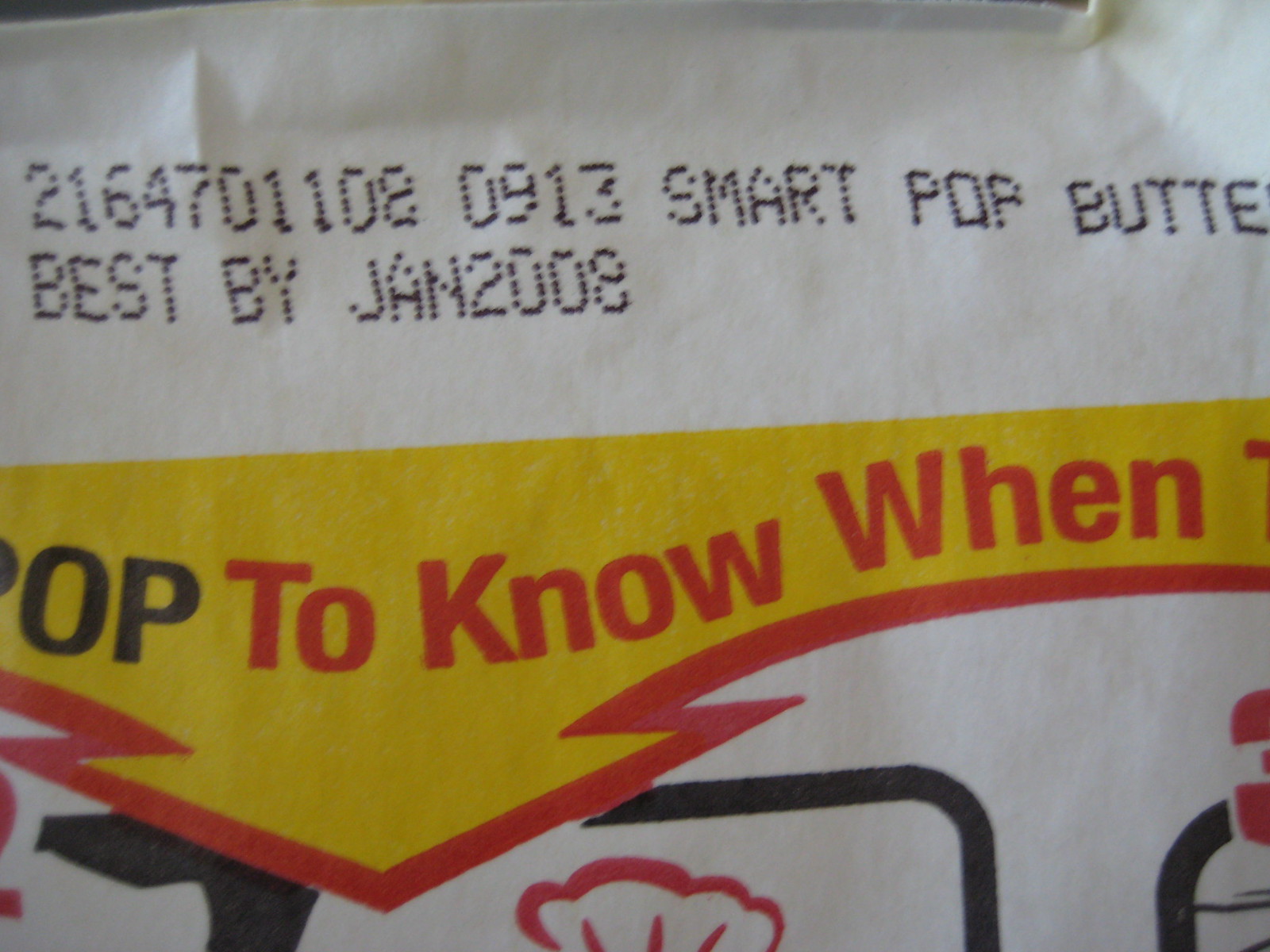The image is a highly detailed close-up photograph of a microwave popcorn package. The visible section includes text that reads "Smart Pop Butter," although the 'R' in "Butter" is partially obscured. Below this text, there is an expiration date that reads "Best By Jan 2008." The close-up nature of the photograph means only a part of the packaging is visible, showing a background in yellow with some black and red text. The text "OP to know when" is discernible, accompanied by a red arrow pointing downward, which seems to form a border around the yellow background. Additional imagery in black and red is present but is too distorted to identify clearly, making it evident that the photo captures only a fragment of the overall package design.